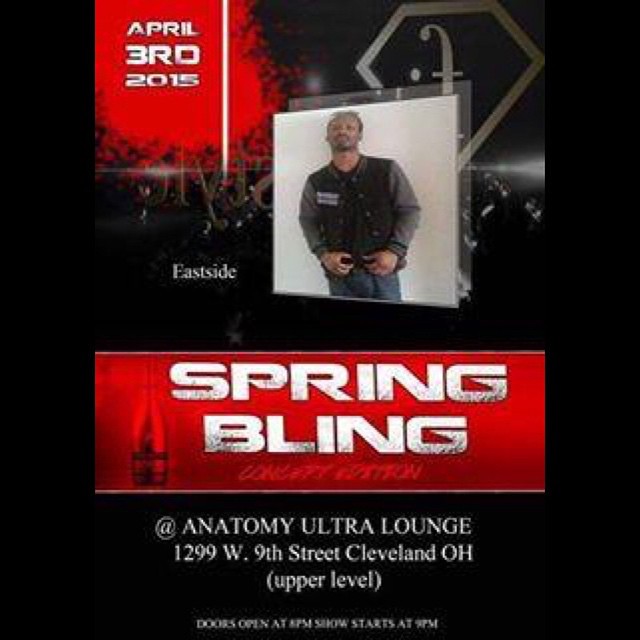The promotional graphic for a nightclub event features a central image of a black man dressed in a black leather jacket with gray sleeves, bluish pants, and a black t-shirt. The backdrop is a blurred scene that could depict a venue with strobe lights and a crowd. To the top left, there's a red circular graphic with gassy effects surrounding it, displaying the date "April 3rd, 2015" in white text. To the top right, a white diamond emblem with a curve-handled sword and a dot can be seen. 

A red rectangular bar below the man's image prominently displays the event's title "Spring Bling," with a washout effect slightly graying the first and last letters. Beneath this bar, the venue's name and details are listed: "Anatomy Ultra Lounge, 1299 W. 9th Street, Cleveland, Ohio (Upper Level)." The image also notes that the doors open at 8 p.m. with the show starting at 9 p.m. The predominant colors in the graphic are black, white, and red.